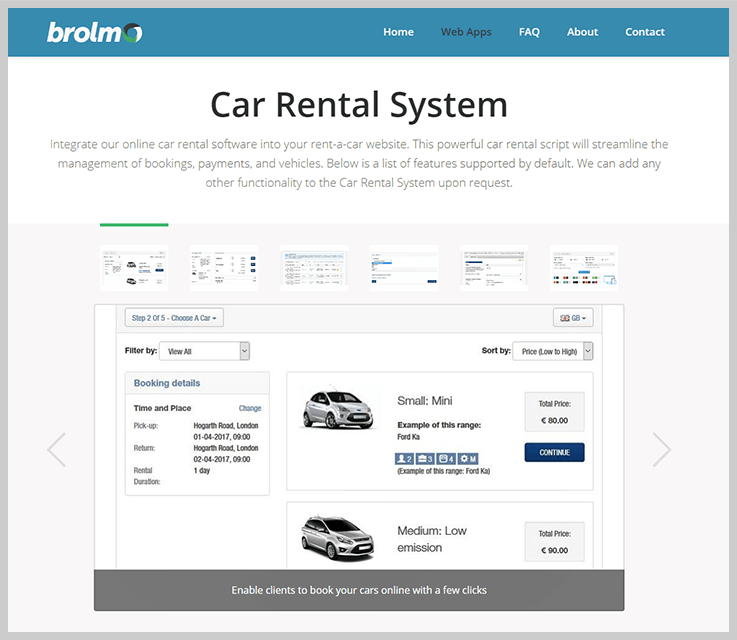This is an image of the Brolem company website. The page features the company's branding, highlighted by a logo in the shape of a circle composed of green, white, and black colors. The company name, "Brolem," is prominently displayed in a teal band that spans horizontally across the top of the page. The entire webpage is outlined in a gray border for a clean and defined look.

Just below the teal band, the navigation menu offers links to "Home," "Web Apps," "FAQ," "About," and "Contact." Dominating the central part of the webpage is a bold headline reading "Car Rental System," with a subheadline inviting users to "Integrate our online car rental software into your rent-a-car website." The accompanying text explains that this powerful car rental script will enhance the management of bookings, payments, and vehicle inventory. It also mentions that additional functionalities can be added to the system upon request.

A green horizontal bar stretches across the page, beneath which are six thumbnail images of different websites, although they are too small to be clearly visible. Below these thumbnails, a larger image showcases a car rental booking interface. The interface allows users to filter and view all booking details, including options for pickup and return times.

The booking options presented feature a small mini car tagged as "medium low emission," priced at $80 with a "Continue" button for proceeding further. Another option for a van, priced at $90, is shown but is cut off, lacking a visible "Continue" button. The section further promotes the ease of online booking with the phrase, "Enable clients to book your cars online with a few clicks."